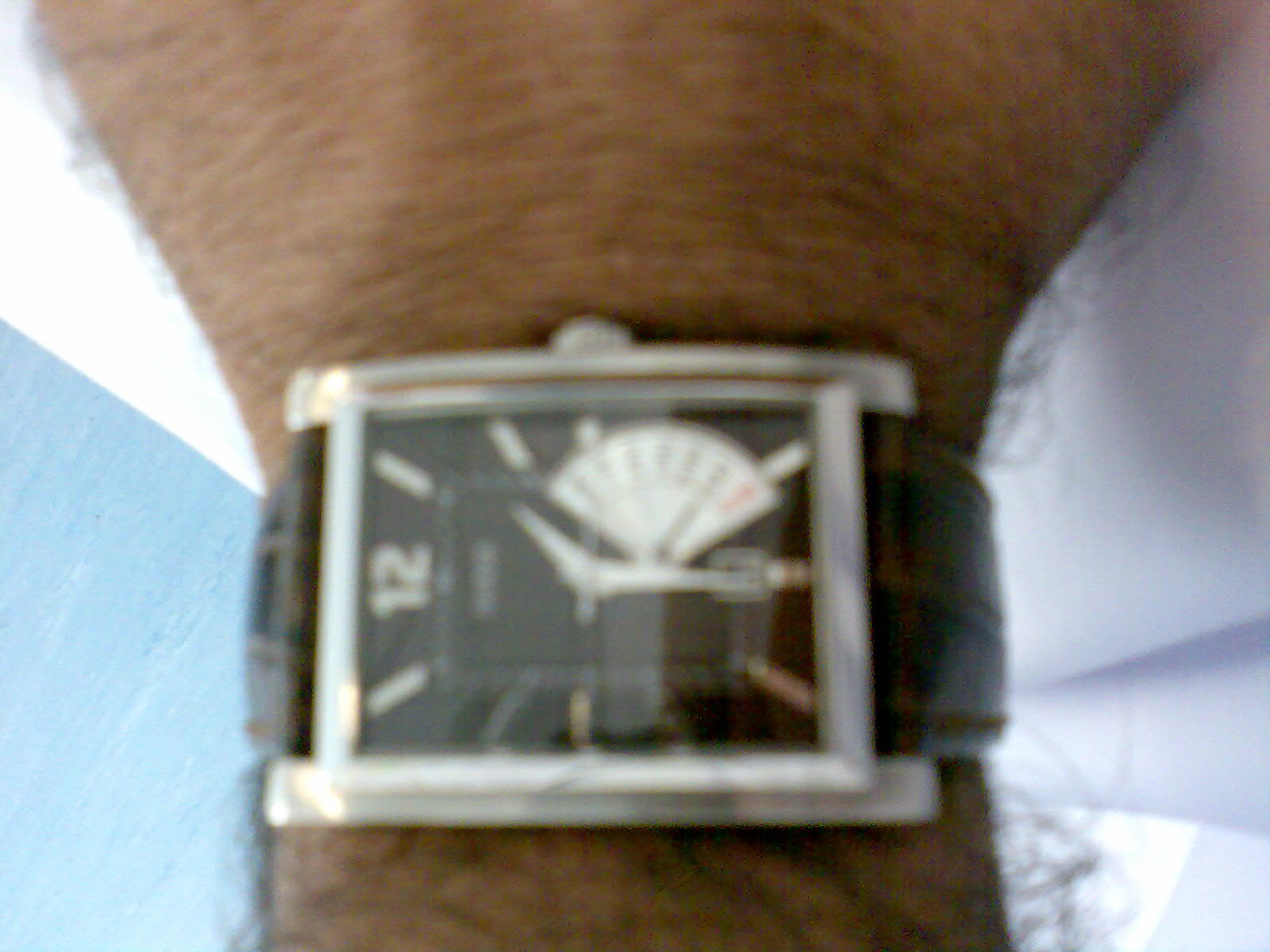The image features a close-up of a man's tanned wrist, adorned with a distinctive wristwatch. The watch, secured by a brown snakeskin band, boasts a sophisticated square face. The dial prominently displays the numbers 12 and 6, while the remaining hour markers are indicated by cream-colored or silver lines. An intricate design resembling a handheld fan with numerical labels is present, with a red numeral situated at the bottom. Although the watch brand name appears on the dial, it is blurry and illegible. The watch includes a spindle for time adjustment, currently indicating the time as 1:30. The man's wrist is resting on a white surface, and there is a noticeable blue color to the left of his hand. His wrist is covered with black hair, adding to the detailed texture of the image.